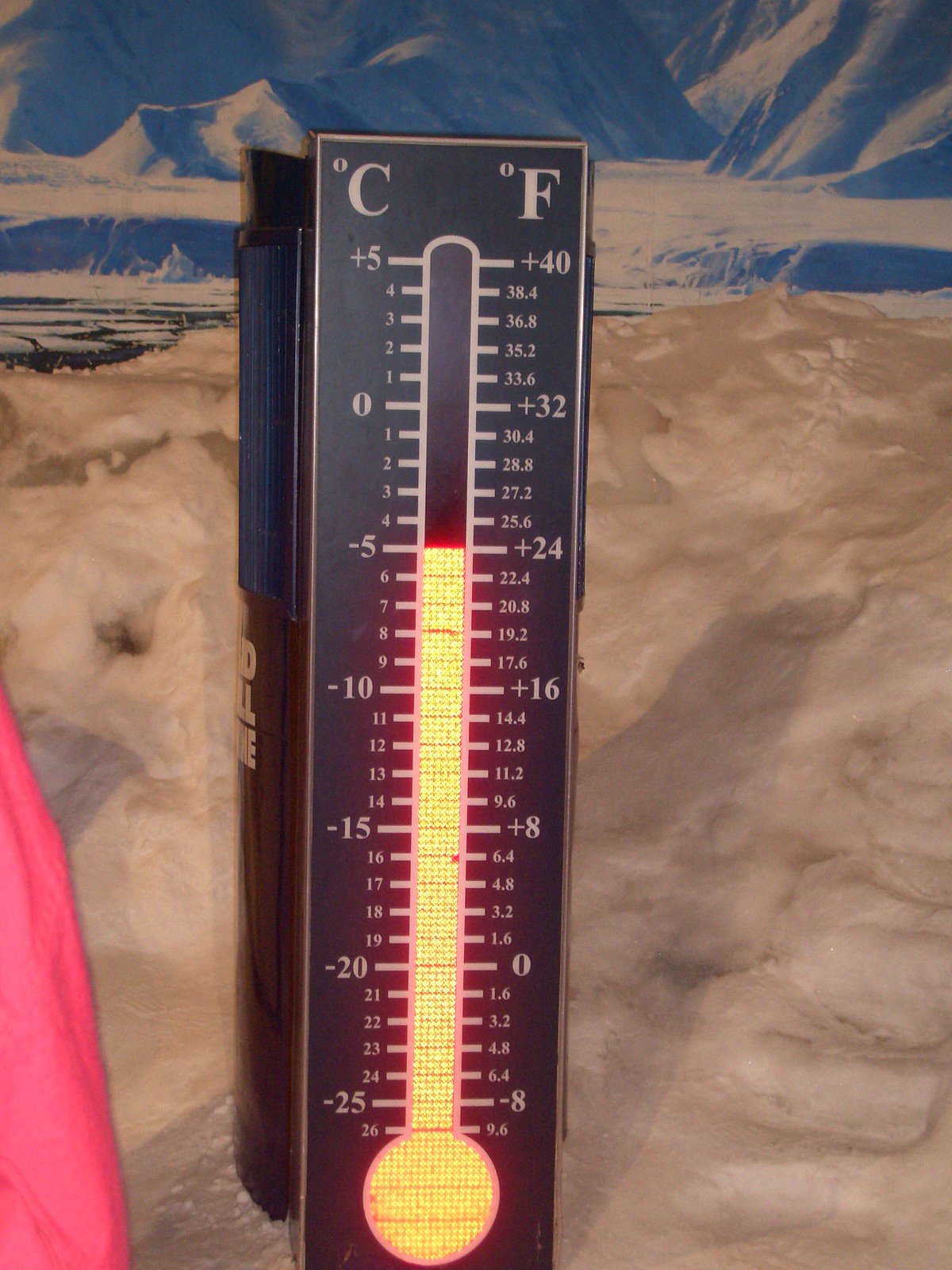The image showcases a black, rectangular thermometer prominently positioned at the center. This thermometer features dual temperature readings in both Celsius and Fahrenheit, marked respectively with a 'C' in the top left-hand corner and an 'F' in the top right-hand corner. The temperature gauge, situated centrally, starts as a circular base at the bottom. Indicated by a yellow light, the gauge spans upward, reaching a range from approximately -5 to +24 degrees.

The background reveals a white, snow-like surface that appears mushy in texture. Above the thermometer, there is a blue area with white markings; the exact nature of this object is unclear, but it appears painted with white hues. To the left side of the image, a soft, pink material resembling clothing is visible, adding a touch of color and texture to the scene.